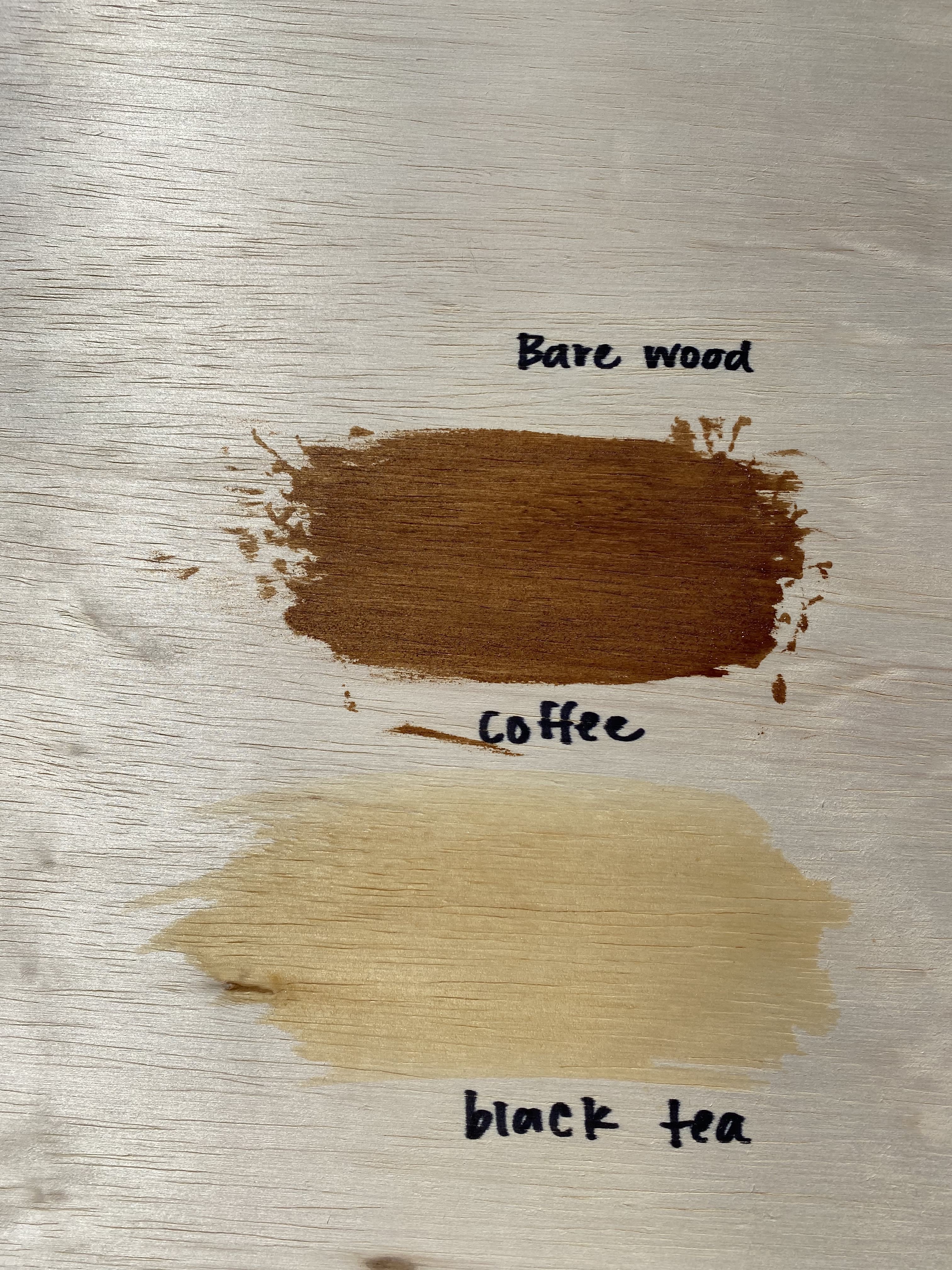The color photo showcases a piece of manufactured, light gray wood with handwritten labels in black sharpie identifying different wood stains. At the top, "bare wood" is written, and beneath it is a dark brown splotch labeled "coffee." This coffee stain appears splotchy with scattered droplets along the edges. Below it is a very light yellowish-brown stain labeled "black tea," which is larger in width but more uniform compared to the coffee stain. The image suffers from some glare, obscuring parts of the wood, but the primary focus remains on the contrast between the dark coffee stain and the paler black tea stain on the washed-out gray background.